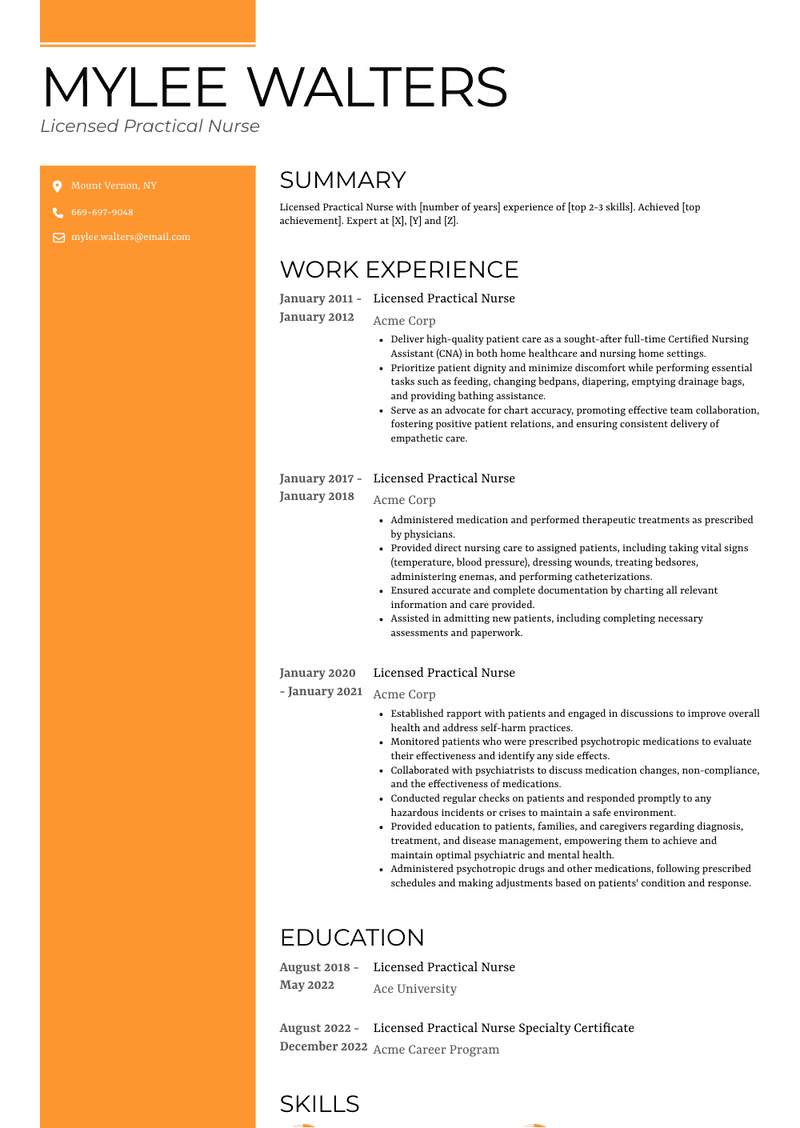This is a detailed screenshot of Miley Walters' resume, who is a Licensed Practical Nurse. The layout features an orange column along the left-hand side, which approximately covers one quarter of the page, and the remaining three-quarters are white with black text. At the top of the orange column is a light orange line, below which Miley Walters' name and title, "Licensed Practical Nurse," are prominently displayed. The column also contains a location marker listing "Mount Vernon, New York," a phone icon next to her phone number, and a mail icon next to her email address. 

The main content of the resume is found in the white section and is organized into several categories. The top section begins with a summary that mentions, albeit the text is too small to read in detail, Miley's years of experience and top skills. This is followed by the "Work Experience" section which details her employment as a Licensed Practical Nurse at Acme Corp over three periods: January 2011 to January 2012, January 2017 to January 2018, and January 2020 to January 2021. Each of these entries includes a list of her responsibilities and accomplishments, although the specific bullet points are too small to discern.

Further down, the "Education" section outlines her academic background, listing her qualification as a Licensed Practical Nurse from Ace University achieved between August 2018 and May 2023, and a specialized certificate from Acme Career Programs for the period from August 2023 to December 2023. The very bottom of the resume, which is partially cut off in the screenshot, seems to list her skills and possibly additional certifications or awards. This structured template provides a comprehensive overview of her professional qualifications and experience.